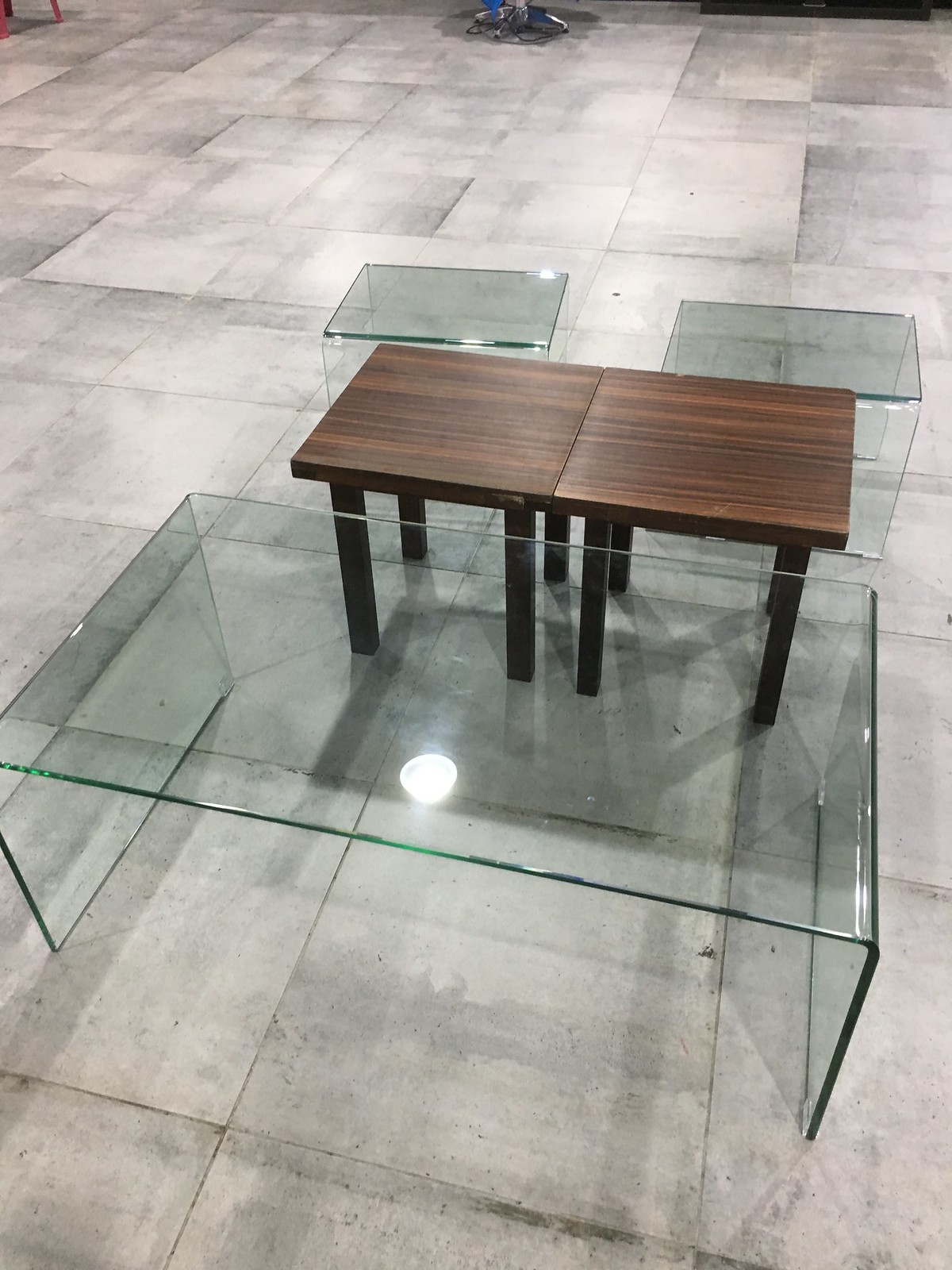The image depicts a collection of tables on a large, tiled concrete floor with grayish-white grout. At the forefront is a sizable glass coffee table, completely transparent with all parts made of glass, including its two leg-like sides. A ceiling light creates a bright glare spot on this table. Next to it sit two smaller glass tables, of the same design but reduced in size. Adjacent to these are two dark wooden tables, placed side by side. These wooden tables can function either as a single coffee table or as separate end tables, and they rest on four legs each. The overall setting from the top-down view highlights the stark contrast between the minimalistic glass tables and the robust wooden ones, all arranged on a neatly tiled surface. A small, unspecified plastic item is also partly visible in the background.